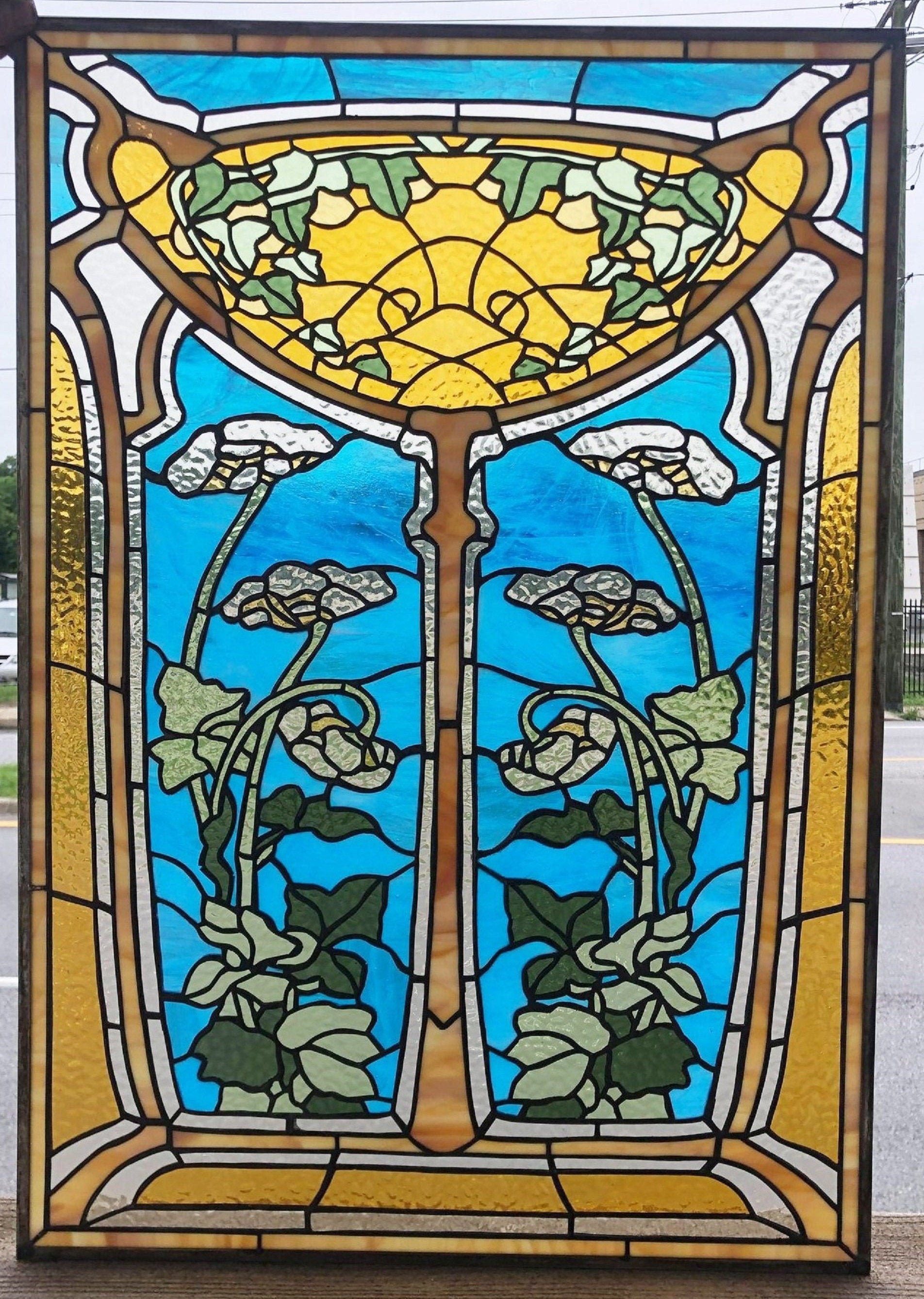This detailed image captures a stained-glass window set against an outdoor backdrop. The window, rectangular in shape and bordered by a dark thin metal frame, rests on a wooden table. The stained glass itself features a striking central design: a large, gold cup-like figure with a long brown handle, transitioning into a bowl-like shape with shades of yellow inside, flanked by flourishing green vines and leaves adorned with white flowers. The background of the glass showcases a serene blue sky, contributing to the window's vibrant and detailed aesthetic. Surrounding this exquisite stained glass is a brown outer border, with gold and silver trim running along its edges. Beyond the window, the outdoor scene reveals a tree-lined street with buildings partly visible on the sides and a fence on the right, hinting at a quaint, leafy neighborhood enveloped in greenery.